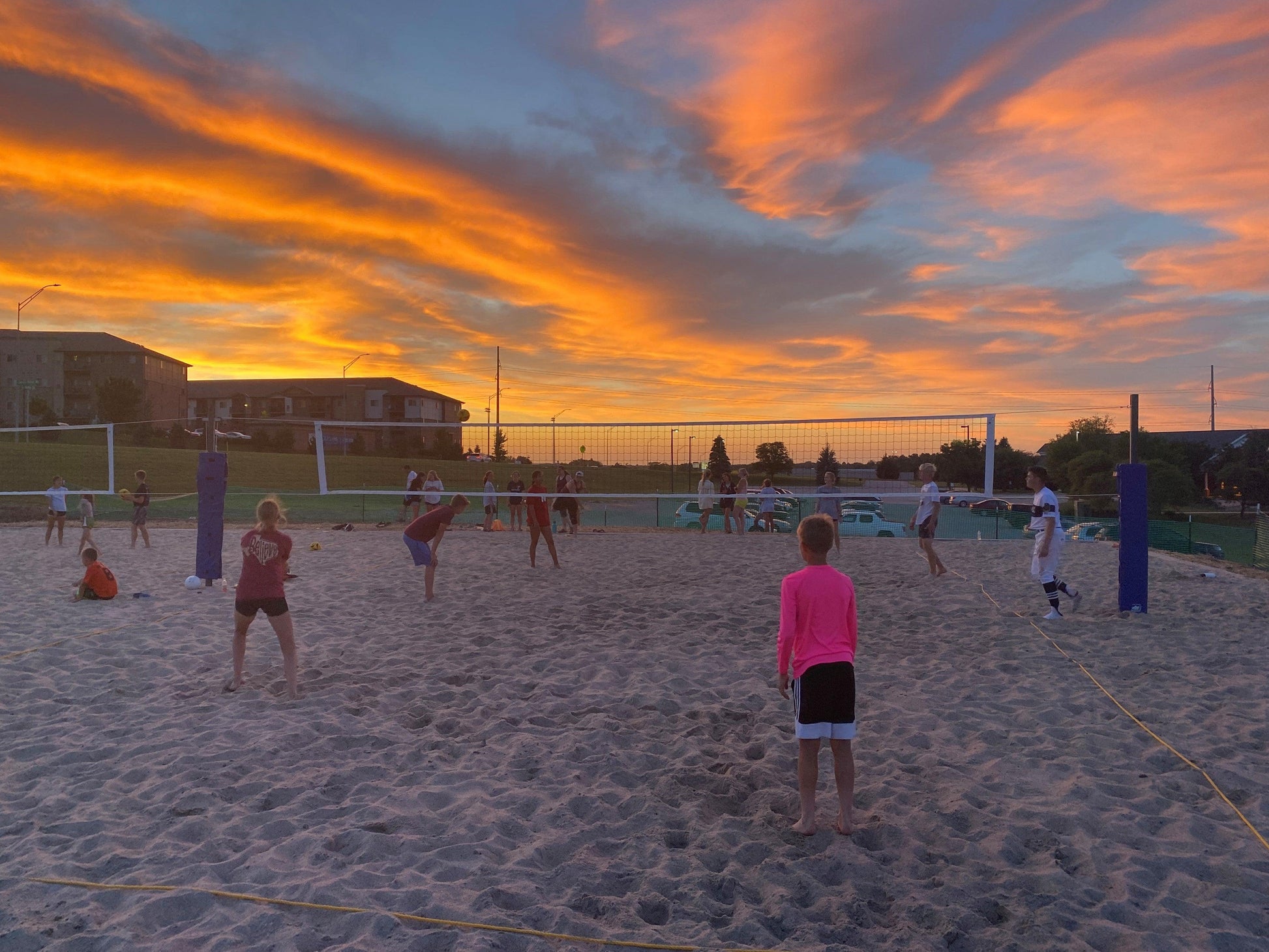In this lively outdoor photograph, a vibrant beach volleyball scene unfolds with two separate courts set up on a sandy area. The foreground features a spirited player closest to the photographer, donned in a bright pink long sleeve shirt and black shorts, poised and ready for the next move. Surrounding the court, a mix of young participants and kids are engaged in the game. To the front and right of the main court, another player with a red shirt and black shorts stands, hair tied back in a ponytail. Behind the nets, a crowded background reveals a parking lot filled with cars and adjacent apartment buildings, under a sky transitioning into the hues of sunset. The sky is thick with clouds, adding to the dusky ambiance. The air is filled with playful energy as the young individuals indulge in the spirited match, with the sandy terrain and makeshift rope boundary lines creating a vivid setting for this friendly sporting event.